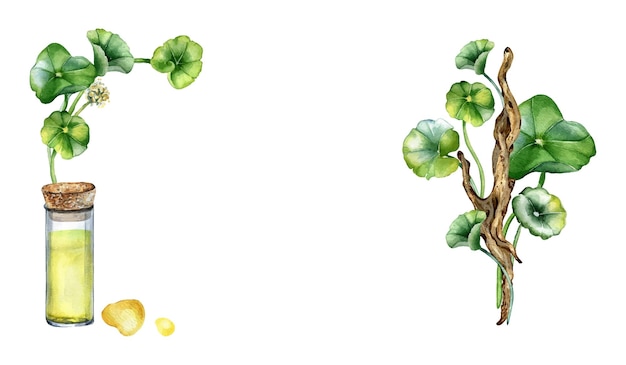This illustration, hand-drawn and water-colored, features two botanical images set against a white background. On the left, a cylindrical glass vial or beaker with a brown cork top contains a yellowish liquid. Emerging from the cork is a long green stem adorned with green and yellow leaves and a budding yellow flower. To the right, there is a depiction of a mature tree branch characterized by a darker brown, wood-like stem. This branch bears larger green and yellow leaves, indicative of a more developed stage of the plant seen in the vial. The detailed illustration appears to serve an educational purpose, potentially from a scientific treatise or textbook, showcasing the growth stages of a certain plant species. The absence of text accentuates the focus on the visual progression from youthful growth in a controlled environment to a mature plant in a natural setting.